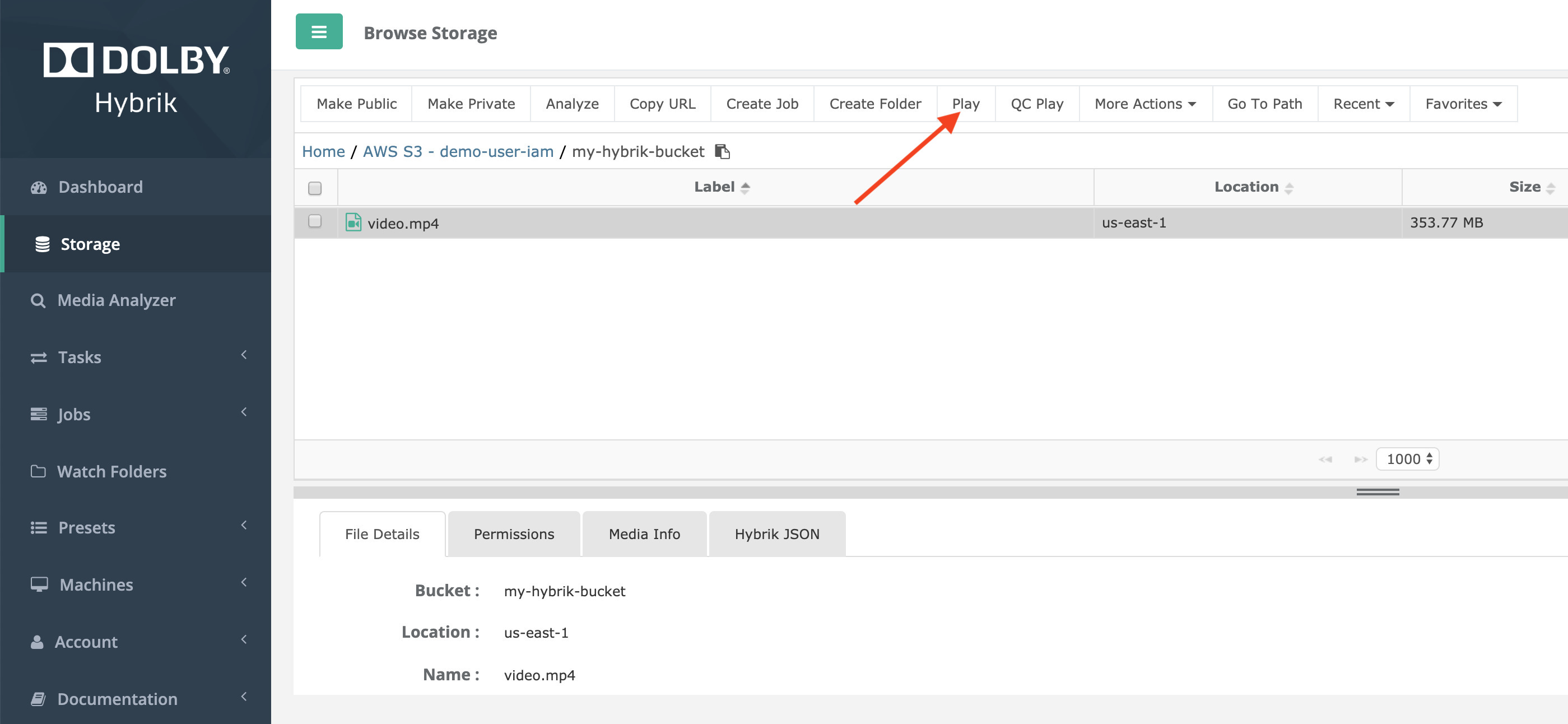The image displays a computer screen in landscape orientation with a detailed user interface.

On the very left side, there's a tall, black panel with a logo and labeled options in block letters. The logo is unclear, but the panel reads "Dolby" followed by "Hybric." Below the logo are several menu options, listed vertically: "Dashboard," "Storage" (highlighted in white, indicating it is currently selected), "Media Analyzer," "Tasks," "Jobs," "Watch Folders," "Presets," "Machines," "Account," and "Documentation." These menu options are mostly in gray text on a black background.

The remainder of the screen is occupied by a white panel. At the top left of this panel, there is a green square containing three white lines, adjacent to dark text that reads "Browse Storage." Directly below this text are several function buttons spread horizontally across the top, from left to right: "Make Public," "Make Private," "Analyze," "Copy URL," "Create Job," "Create Folder," "Play," "QC Play," "More Actions," "Go-To Path," "Recent," and "Favorites." Notably, a red, hand-drawn arrow points toward the "Play" button, starting from below and left, with its arrowhead touching the bottom left of the "Play" button.

Below the function buttons is a navigation path displaying "Home / AWS S3 Demo User LAM / MyHybricBucket." Underneath this, a single file, "Video.mp4," is highlighted in a gray row. Above this row are column headers: "Label," "Location," and "Size." The selected file has the following details in the row: Label as "Video.mp4," Location as "US East 1," and Size as "353.77 MB."

Further down, the screen features a large white space, and near the bottom are four tabs in a row: "File Details" (selected and shown in white), "Permissions," "Media Info," and "Hybrid JSON" (all in gray). The "File Details" tab displays specific information for the selected file, including Bucket, Location, and Name.